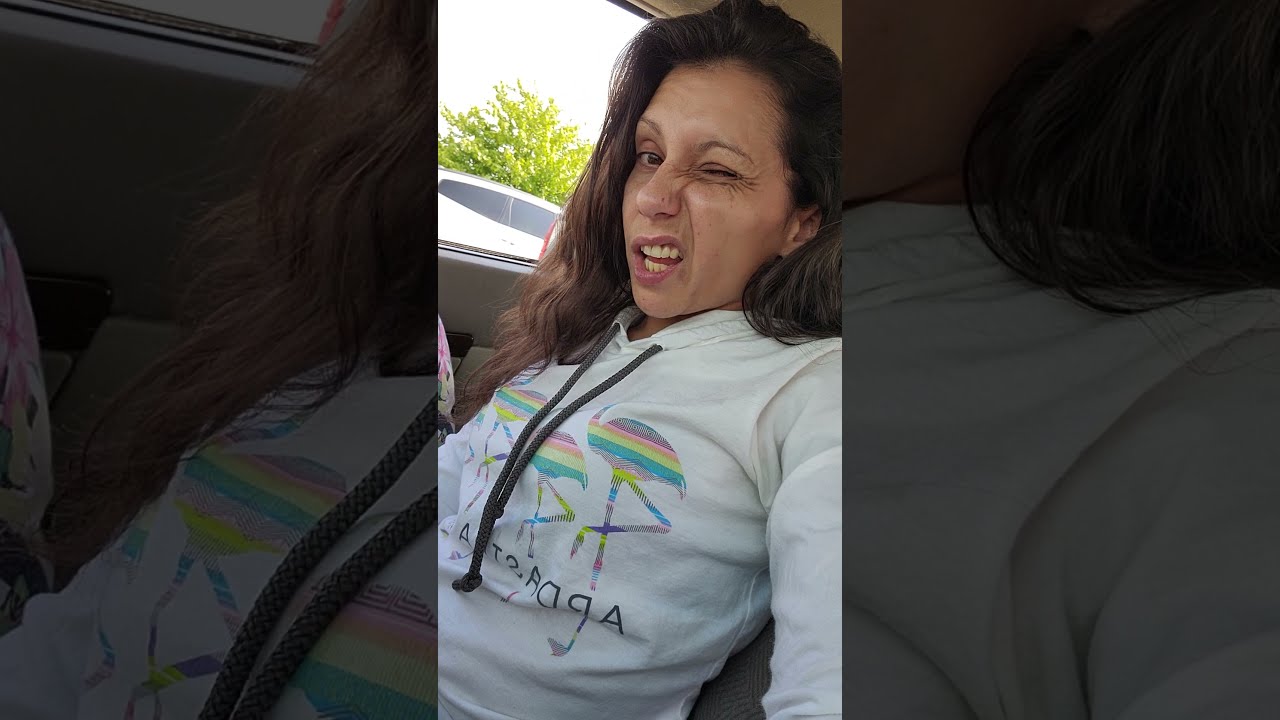The photograph captures a woman sitting in the front passenger seat of a car. She has long brown hair that is parted to the far side from the camera, revealing her right eye which is open, while her left eye is closed in an attempt to wink. Her expression shows her mouth open, displaying both sets of teeth, and the left side of her face is scrunched upward. She is wearing a white hoodie with gray drawstrings, decorated with colorful flamingos in stripes of purple, pink, yellow, and blue. Although there is lettering beneath the flamingos, it is illegible. The car's interior is a tannish color. Out the car window, a tree and another vehicle are visible under a brightly lit sky. The composition is unique, featuring not only the central image of the woman but also shaded, enlarged versions of the same photo on both the left and right sides, with a close-up of the flamingos on her shirt on the left.